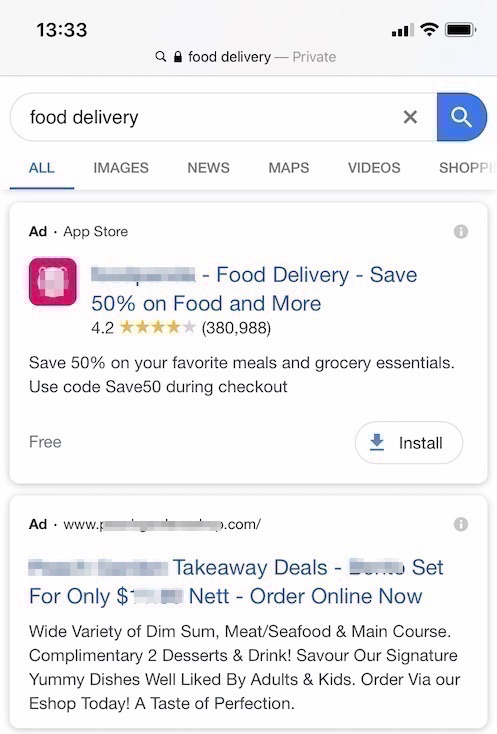The image displays a food delivery search on a mobile phone at 13:33, as indicated by the military time format. The phone shows a full battery and a Wi-Fi connection. The search for food delivery is labeled as locked and private. Below the search bar, there are tabs for "All," "Images," "News," "Maps," "Video," and "Shopping." 

An advertisement is prominently displayed, promoting a food delivery app available from the app store. Although the app's name is redacted, the ad boasts a notable offer: save 50% on food and grocery essentials by using the code SAVE50 at checkout. The app has a rating of 4.2 stars from approximately 380,000 reviews. The app is free to install.

Another advertisement, with the website name redacted, promotes takeaway deals with a placeholder for the price, indicating there are special deals available. The ad highlights a wide variety of dishes, including dim sum, meat, seafood, and main courses, along with complimentary desserts and drinks. It emphasizes the variety and appeal of their signature dishes, which are enjoyed by both adults and kids.